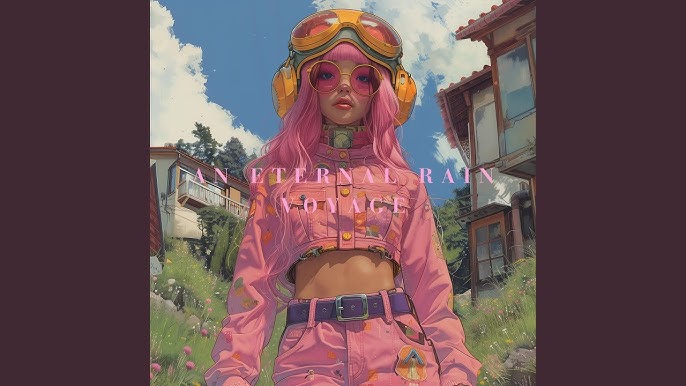In this computer-generated, highly realistic image, a young, fair-skinned girl stands in the foreground of a vivid outdoor setting. The backdrop is a clear blue sky decorated with soft, puffy white clouds, flanked by two-story houses; one prominently visible on the right with a partially seen upper-level railing, and another, more worn-looking structure, suggesting a different country. The scene is enclosed by thick, vertically-aligned, dark purple borders on either side.

The girl has striking wavy, long hot pink hair with bangs that fall on her forehead, and she wears large, round pink-tinted glasses. Resting atop her head are large yellow goggles and yellow over-ear headphones. Her outfit is equally eye-catching, featuring a colorful crop-top jacket adorned with a pattern that might depict food items, ending above her exposed midriff and paired with pink pants fastened with a purple belt.

She stands amidst a grassy area with scattered flowers, embodying a whimsical and vivid fashion aesthetic. Across her chest area, the text "An eternal rain voyage" is printed in light pink letters, adding a final touch of intrigue to this arrestingly detailed visual narrative.